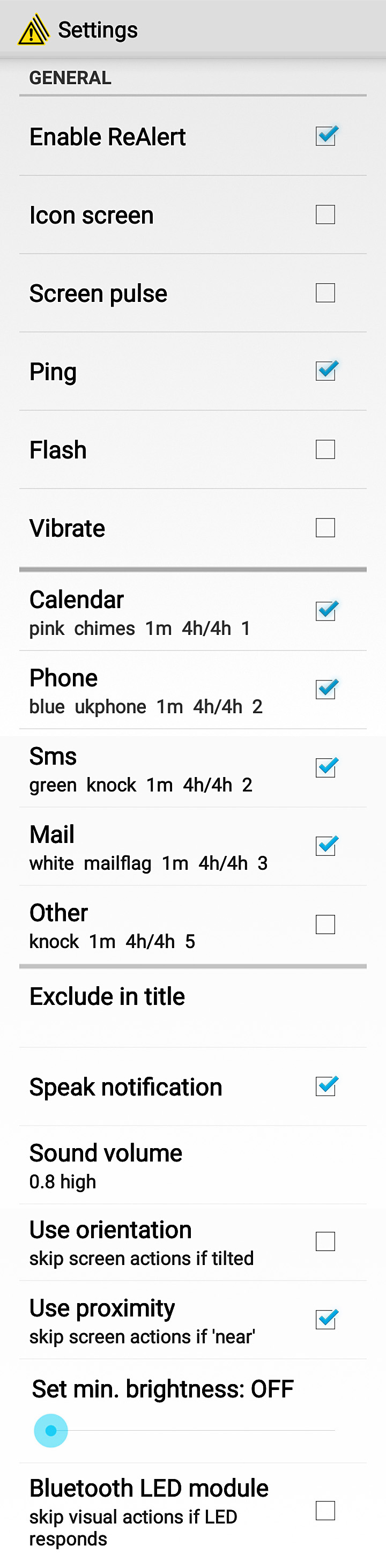The setup under the "Websites" section is evidently cramped into a space that's too limited for it, causing the text to appear squashed. An alert is displayed, with "Settings" indicated underneath. Within the settings menu, the "General" tab is selected, showing the following options and their statuses:

- **Enable Alert**: Checked
- **Icon Screen**: Not checked
- **Screen Pulse**: Not checked
- **Ping**: Checked
- **Flash**: Not checked
- **Vibrate**: Not checked

**Calendar Notifications:**
- **Sound**: Pink Chimes
- **Duration**: 1 minute
- **Status**: Checked

**Phone Notifications:**
- **Sound**: Blue
- **Region**: UK
- **Duration**: 1 minute
- **Status**: Checked

**SMS Notifications:**
- **Sound**: Green Knock
- **Duration**: 1 minute
- **Status**: Checked

**Mail Notifications:**
- **Sound**: White Mail Flag
- **Duration**: 1 minute
- **Status**: Checked

**Other Notifications:**
- **Sound**: Knock
- **Status**: Not checked

Additional Settings:
- **Exclude in Title**: Not checked
- **Speak Notification**: Checked
- **Sound Volume**: 0.8 (High)
- **Use Orientation**: Not checked
- **Skip Screen Action if Tilted**: Indicated but not checked
- **Proximity Sensor**: Checked
- **Skip Screen Actions if Near**: Indicated
- **Set Minimum Brightness**: Off